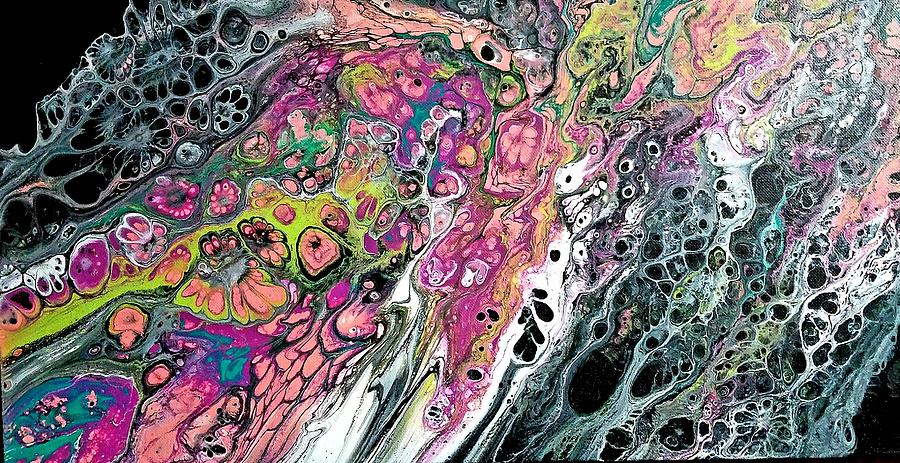This horizontally oriented abstract artwork features a vibrant, multicolored display set against a black background, resembling a stunning combination of watercolor and digital painting techniques. The image bursts with a multitude of shapes that evoke the appearance of running water interspersed with bubbles and seafoam. Dominant on the left side are vibrant hues such as intense yellow, fuchsia, blue, and teal, creating a striking contrast with the more subdued, washed-out tones of whites, greens, and grays on the right. The piece is filled with swirling and circular patterns, reminiscent of microscopic cellular structures or the intricate designs formed by paint or oil suspended in water. Throughout, the interplay of colors—ranging from pinks and peaches to blues and greens—along with the abstract, randomized feel of the composition, makes the artwork both colorful and captivating.